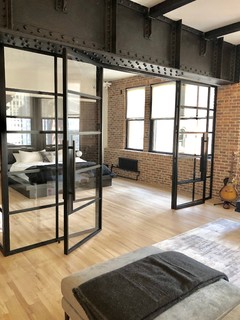The photograph captures the interior of a modern apartment, showcasing a clean, contemporary design. Dominating the center of the vertical frame are large glass double doors, bordered by dark horizontal and vertical lines. These doors lead into a bedroom where a queen or king-sized bed, neatly made with pillows and a dark blanket, is visible. Adjacent to the bed is a textured brick wall, punctuated by three separate windows allowing natural light to filter through. The ceiling within the space contrasts starkly in white, while a substantial horizontal dark wood or black beam accentuates the entryway to the bedroom. In the foreground, a white and gray area rug occupies the lower right corner near an ottoman draped with a blanket or towel. A light brown wood tile floor runs throughout, adding warmth to the room's monochromatic palette of blacks, whites, grays, and touches of beige and tan. A guitar and stand are subtly positioned beside the windows, further enhancing the room's modern yet cozy ambiance.